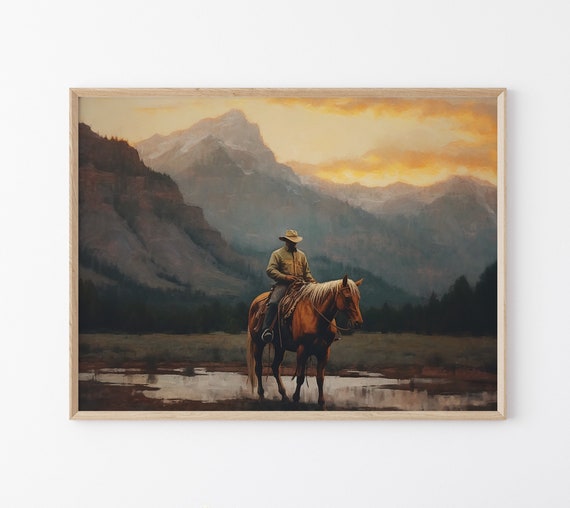The image showcases a framed piece of artwork with a meticulously crafted wooden rectangular frame. The artwork is a highly realistic painting depicting a cowboy or a man adorned in a cowboy hat, a tan long-sleeved jacket, and blue jeans, confidently riding a magnificent brown stallion with flowing blonde mane. The horse is gracefully stepping through a small puddle, surrounded by a lush meadow of verdant grass. In the background, a majestic mountain range towers, bathed in the golden-orange hues of a breathtaking sunset. A row of trees lines the base of the mountains, adding depth and tranquility to the scene. This idyllic portrayal captures the serene beauty of nature and the rugged elegance of the cowboy's journey.